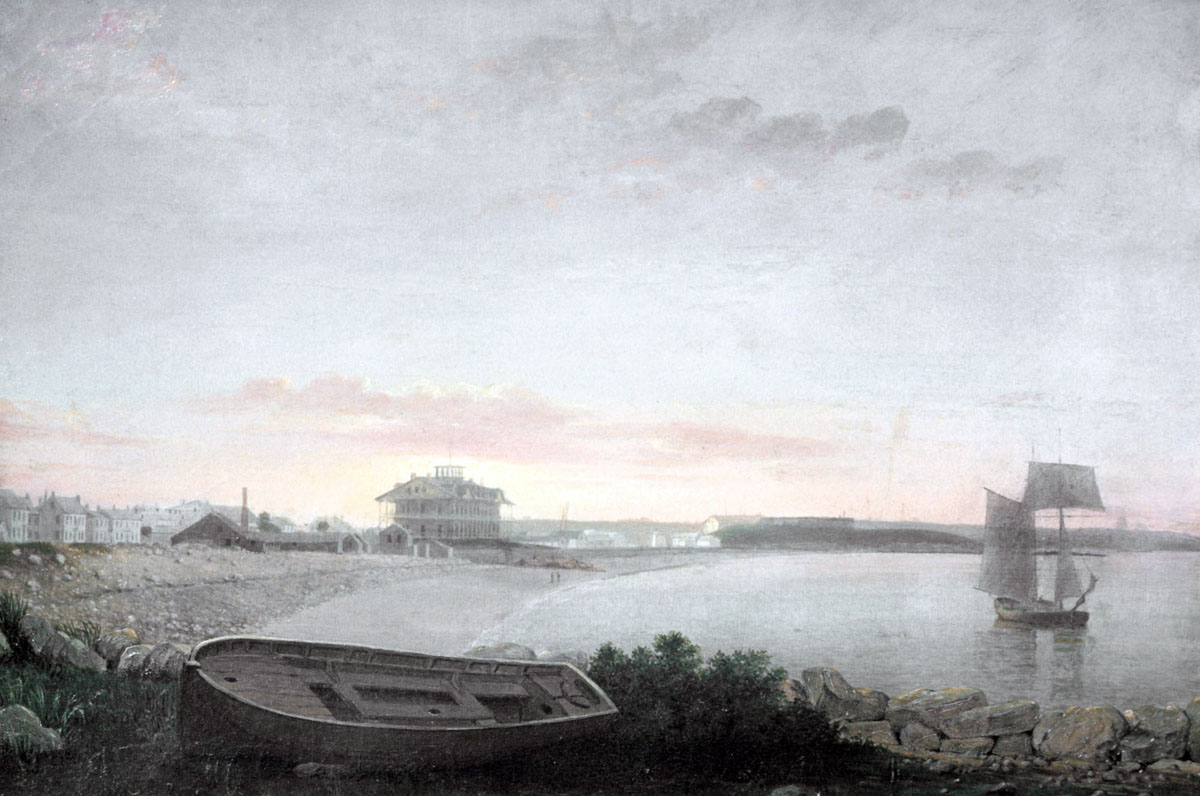In this detailed painting of an ocean scape, an old-timey sailboat with its sails unfurled navigates the waters in the bay, situated towards the middle right of the image. The craft's historical design stands out against the backdrop of choppy, pink-tinged gray skies, indicating imminent weather changes. On the left side of the picture, there's another boat, an old rowboat, situated on the sandy beach, positioned at the lower-left corner with its bow facing left, leaning slightly towards the viewer. This boat is depicted in a gray-brown hue, clearly detailed.

The shore is lined with big rocks, especially prominent in the bottom right corner where they are piled high, creating a rugged boundary. Along the beach, there's a protective bank structure, presumably to prevent flooding, which adds a layer of realism to the scene. Scattered bushes add a touch of greenery, most notably a dark-colored one adjacent to the beached rowboat.

In the background, the painting captures a small beach community featuring a variety of buildings. The left middle section of the image showcases these structures, including a prominent three-story building among smaller one- and two-story houses. The buildings, painted in muted tones, appear slightly blurred by the atmospheric conditions, with the tallest placed near the seashore. This community, extending towards the horizon, complements the lively seascape below and harmonizes with the moody sky above.